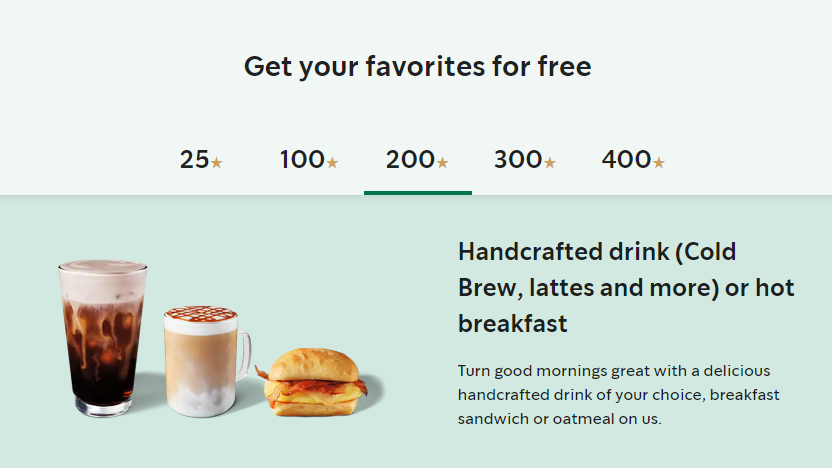The webpage displays a promotional section for Starbucks Rewards, prominently positioned at the top center with the message, "Get your favorites for free," in bold black text. Beneath this headline, a tiered points system is outlined:

- **25 points** - Represented by the number "25" next to a small gold star.
- **100 points** - Represented by the number "100" next to a small gold star.
- **200 points** - Represented by the number "200" next to a small gold star.
- **300 points** - Represented by the number "300" next to a small gold star.
- **400 points** - Represented by the number "400" next to a small gold star.

Underneath the "200 points" label, a green bar highlights this tier, indicating it’s currently selected. The right side of this section elaborates on the rewards available at 200 points, stating: "Receive a handcrafted drink, cold brew, lattes, and more, or a hot breakfast." Further details explain, "Turn good mornings great with a delicious handcrafted drink of your choice, breakfast sandwich, or oatmeal on us."

To the left of this text, and below the "25 points" section, there are visual depictions of rewards:
- A cold brew latte in a glass.
- A caramel macchiato in a cup.
- A breakfast sandwich positioned to the right of the beverages.